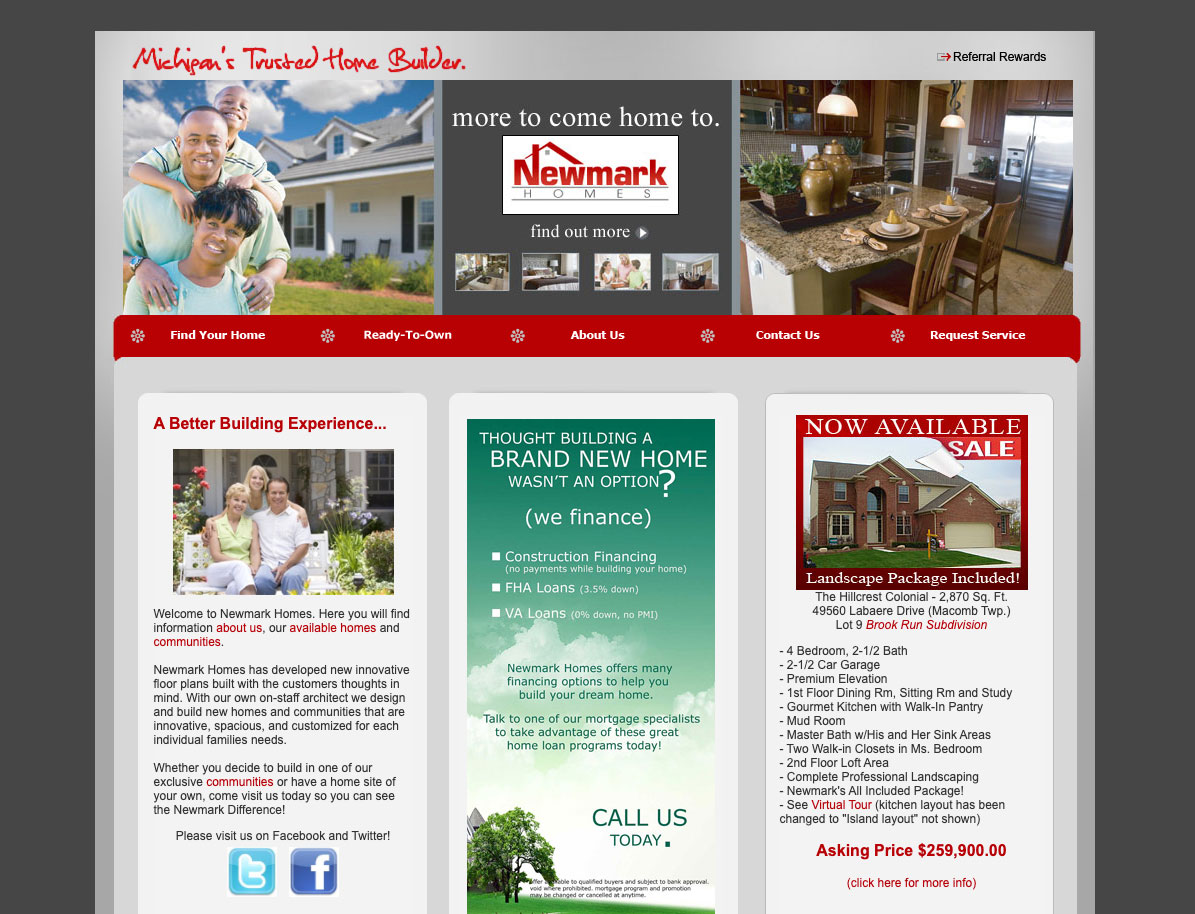Screenshot of a web page featuring a prominent border of dark grey around the left, right, and top sections. Below the border, there's a light grey bar with the phrase "Michigan's Trusted Home Builder" written in elegant red cursive font. In the upper right corner of this bar, "Referral Rewards" is displayed in black font. Below the bar, the content is divided into three sections. The left section shows an image of a happy African American family: a woman with short hair, a taller man resting his hands on her shoulders, and a seven-year-old child hugging the man's shoulders. They stand in front of a picturesque suburban home with a white picket fence. The center section features a dark grey square with white text that reads "More to Come Home to Newmark Homes. Find Out More." The right section showcases a high-end kitchen, complete with a marble island and two wooden chairs. A meticulously set breakfast is placed on the island, including delicate egg cups holding boiled eggs.